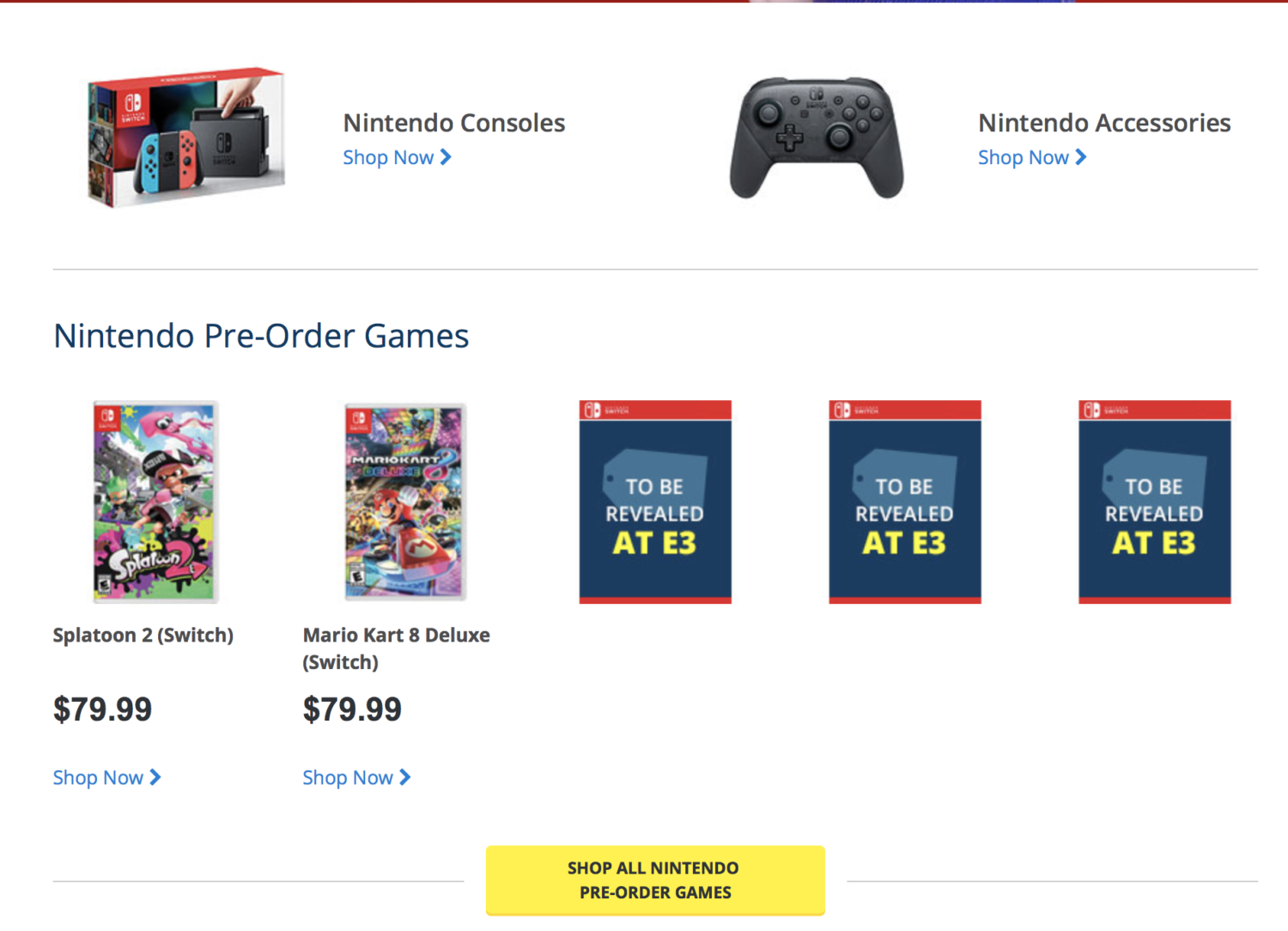This vibrant screenshot is from an unspecified web page, featuring sections dedicated to Nintendo products. In the top-left corner, a banner reads "Nintendo Consoles - Shop Now." Adjacent to this text, a photograph of the Nintendo Switch packaging is displayed. The box prominently features the words "Nintendo Switch" and showcases a hand interacting with the sleek black console. The packaging highlights the distinctive Joy-Con controllers, with the left one in blue and the right one in red.

Directly below, there is an image of a black Nintendo game controller, accompanied by the text "Nintendo Accessories - Shop Now." Further down, the section labeled "Nintendo Pre-Order Games" displays cover art for upcoming titles. The box art for "Splatoon 2" for the Switch is priced at $79.99, followed by the cover art for "Mario Kart 8 Deluxe" for the same price. Additionally, three placeholders with the message "To be revealed at E3" tease future releases. At the bottom of the screenshot, a striking yellow rectangle with black text invites users to "Shop All Nintendo Pre-Order Games."

Absent of any human figures or buildings, the focus of this screenshot is solely on showcasing Nintendo products and their exciting offerings.